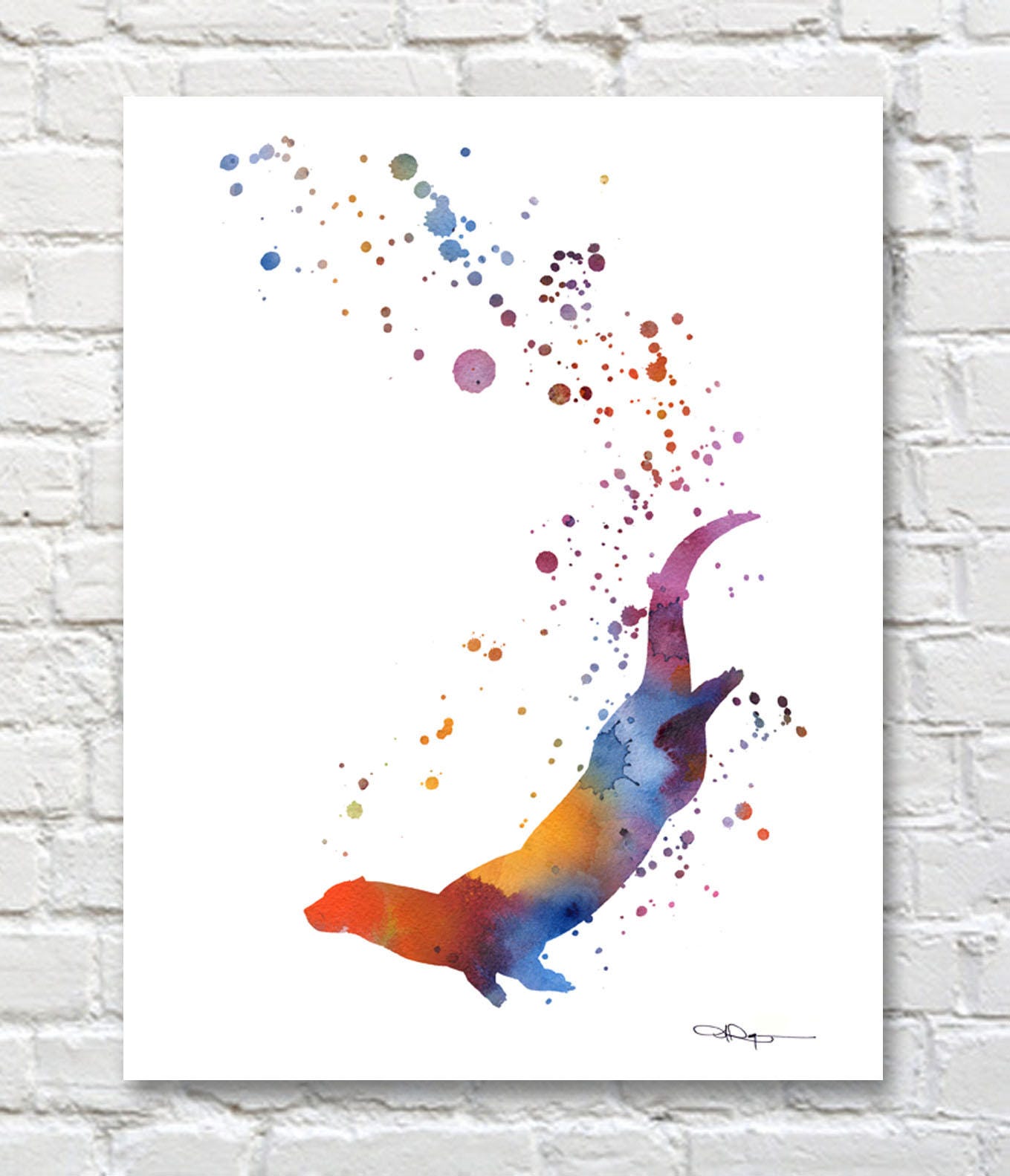Hanging on a light gray brick wall is an abstract watercolor painting on a vertical white canvas. The central subject of the painting appears to be a sea animal, likely an otter, depicted in vivid hues. The otter is portrayed swimming downward, with its red head transitioning into an orange neck, a yellow body with a blue underbelly, and blue front legs. Its back legs are purple, leading into a lighter purple, upward-curving tail that eventually curves downward. Surrounding the otter are variously sized and colored circular dots, resembling air bubbles. The image is framed by a thin border of the white-painted brick wall, emphasizing the canvas. At the bottom right corner of the painting, there is a signature, presumably from the artist. This use of color and composition suggest a deliberate blending and dripping technique, much like watercolor, with defined edges perhaps achieved through stencil application.